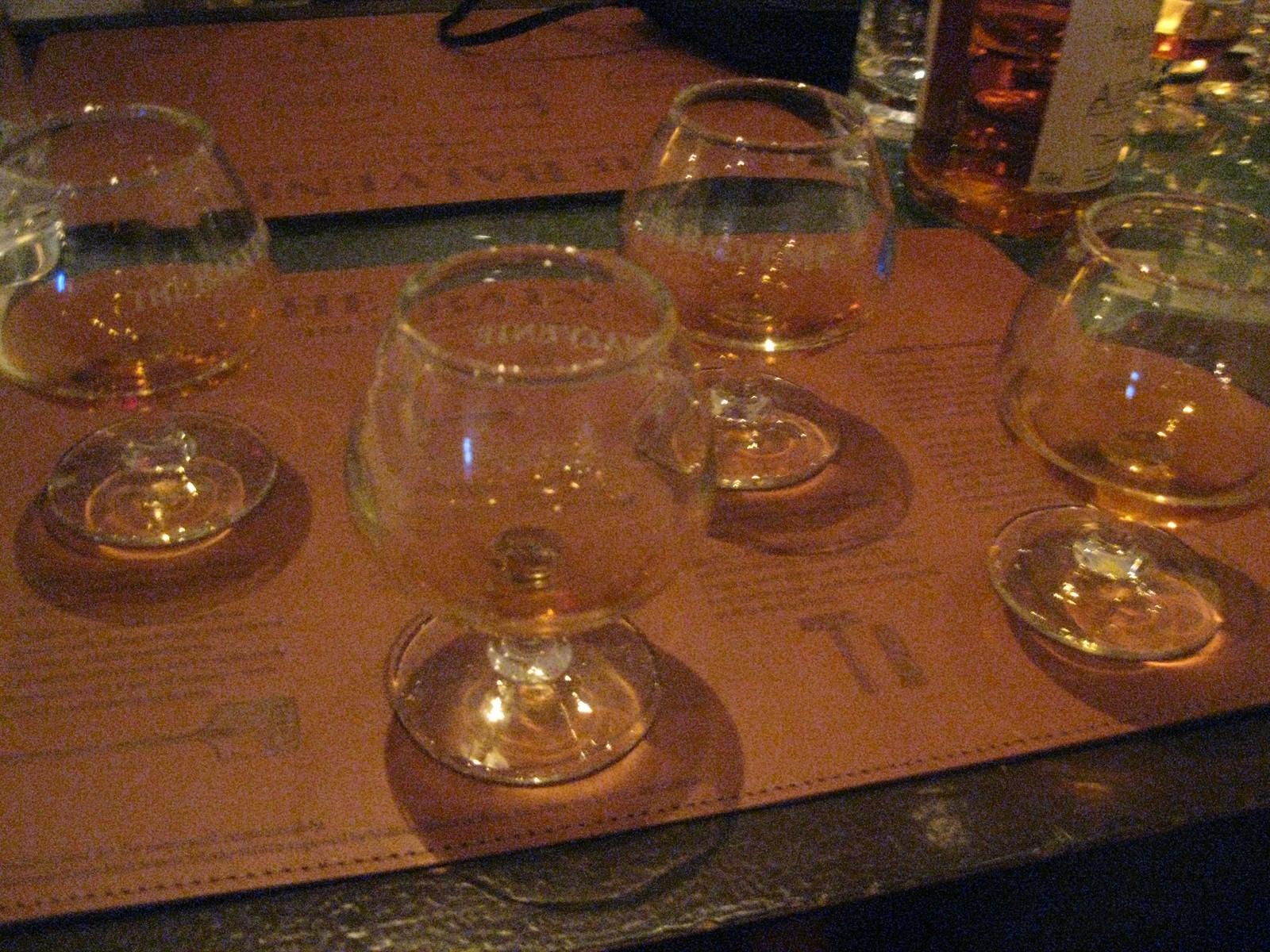The image depicts a wine tasting setup featuring four clear, short-stemmed glasses, commonly used for bourbon, arranged in a zigzag pattern across a brown, leather-like placemat positioned atop a grayish, dark-colored table. The glasses have wide, rounded bases tapering into shorter necks, creating a curved cylindrical shape. Each glass is empty, and they are sporadically placed on the placemat, which is adorned with unreadable text. Behind the primary placemat is another similar mat, a few inches away. In the background, there is a bottle of alcohol with illegible writing on it, and additional glasses are visible. The scene is set in a dimly-lit, relaxed environment, enhancing the cozy ambiance of the wine tasting experience.